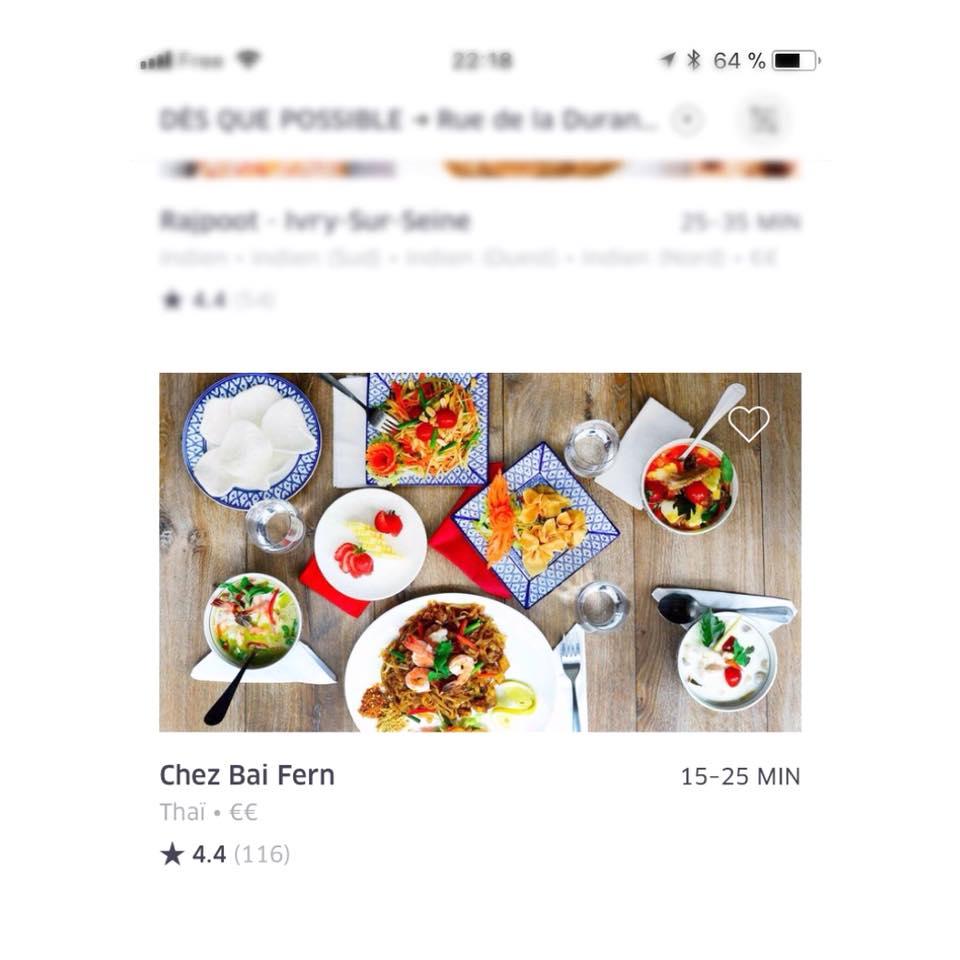A screenshot from a mobile phone, possibly taken from a recipe site or a restaurant app, shows a blurred section at the top with visible indicators of mobile service and a 64% battery level. The blurred text near the top reveals partial letters "D-E-S-K-Q-U-E." Below the blurred text, a vibrant image showcases a variety of dishes presented on several plates and bowls of different shapes and colors, including blue and white, square and round, emphasizing the diversity of the offerings. Below the food image, the restaurant name "Chez Baifern" is displayed prominently, noted to be 15 to 25 minutes away. The restaurant, which specializes in Thai cuisine, boasts a 4.4-star rating based on 116 reviews.